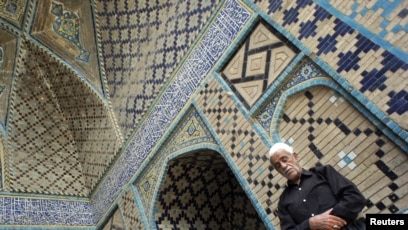The photograph depicts the intricate interior of what appears to be a mosque, captured from a near-ground, slightly tilted perspective. The walls are adorned with vibrant mosaic tiles, displaying a variety of colors and patterns including green, blue, black, brown, and cream. The ceiling is equally elaborate, contributing to the overall ornate design of the building. In the bottom right corner of the image, the word "Reuters" is printed in white letters on a small black panel.

Standing in the bottom right section of the photograph is a man with a darker skin complexion and short white hair, dressed in a long-sleeved black button-down shirt with white buttons. His hands are folded and resting on his stomach, and his eyes are closed, suggesting that he is praying. The overall scene is bright and clear, thanks to natural lighting that highlights the detailed craftsmanship of the interior.